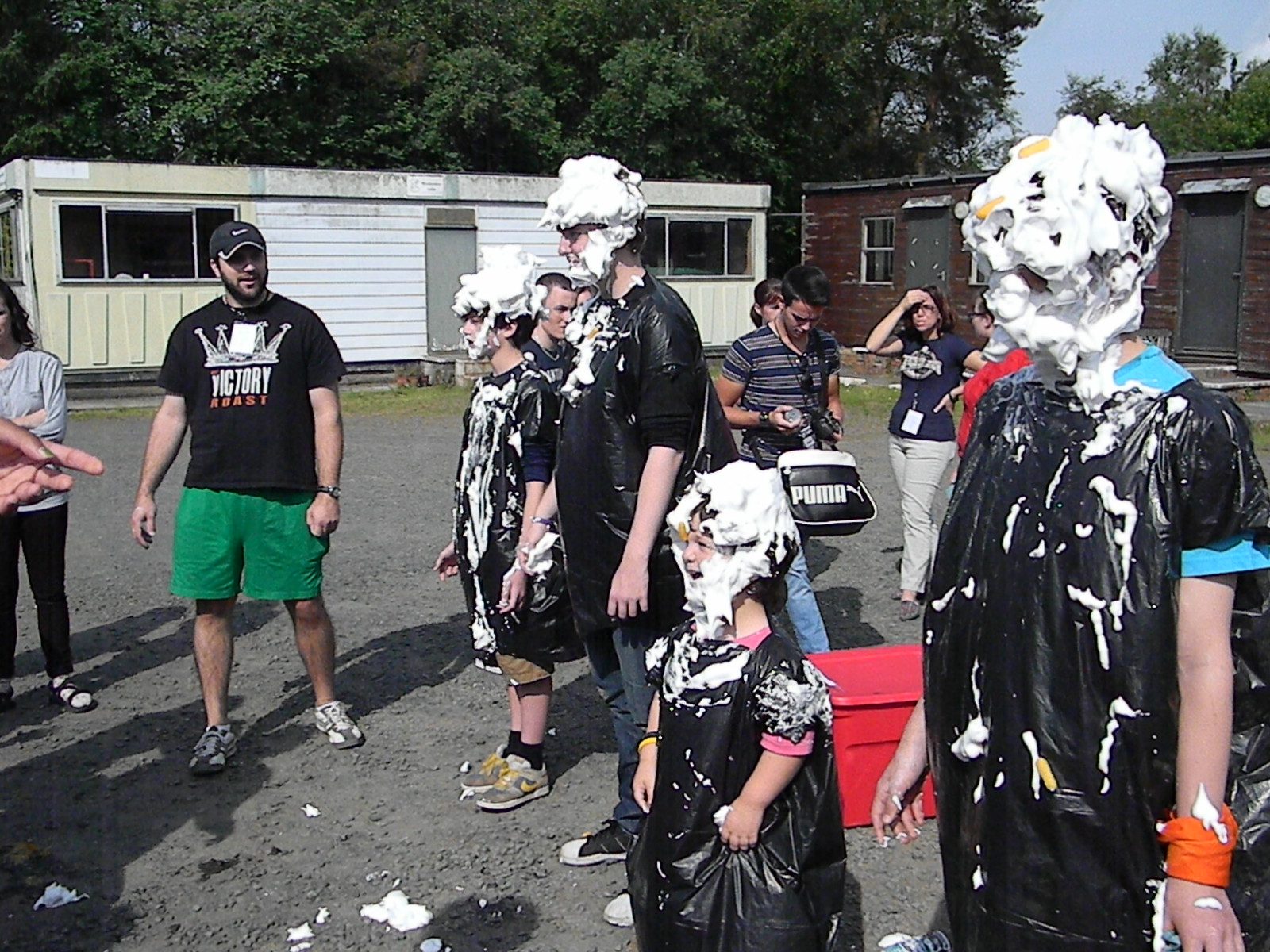In the center of the image, there are four people covered in what appears to be thick, sudsy shaving cream, wearing makeshift smocks fashioned out of black garbage bags with holes cut for their heads. The group consists of two young boys on the edges, a man second from the left, and a little girl, identifiable by a glimpse of her pink shirt beneath the cream, in the third position from the left. To their left stands a man wearing a black Nike cap, a black T-shirt emblazoned with "Victory Roast" and a crown, green shorts, and running shoes. He looks amused, a piece of white paper possibly hanging from his neck. Partially visible to his left is a woman in Birkenstock-style sandals with socks, black pants, and a long-sleeved gray shirt. Further in the background are six additional people, appearing mostly young, with one wearing a blue and gray striped shirt and carrying a black Puma bag, and another in a blue shirt with khaki pants.

The setting features two trailer-like buildings in the background: one on the left with yellow walls and a white door, and another in disrepair with peeling reddish-brown siding and a couple of gray doors on the right. A massive tree occupies much of the background space. The event, likely a community or charity gathering, takes place in a sunny, gravel parking lot, where spectators — with one visibly amused and others glancing away — are gathered around, observing the scene. A large red plastic tote box is seen on the ground among the participants. The overall atmosphere suggests a playful, community-centered activity where participants and onlookers are immersed in the event's lightheartedness.